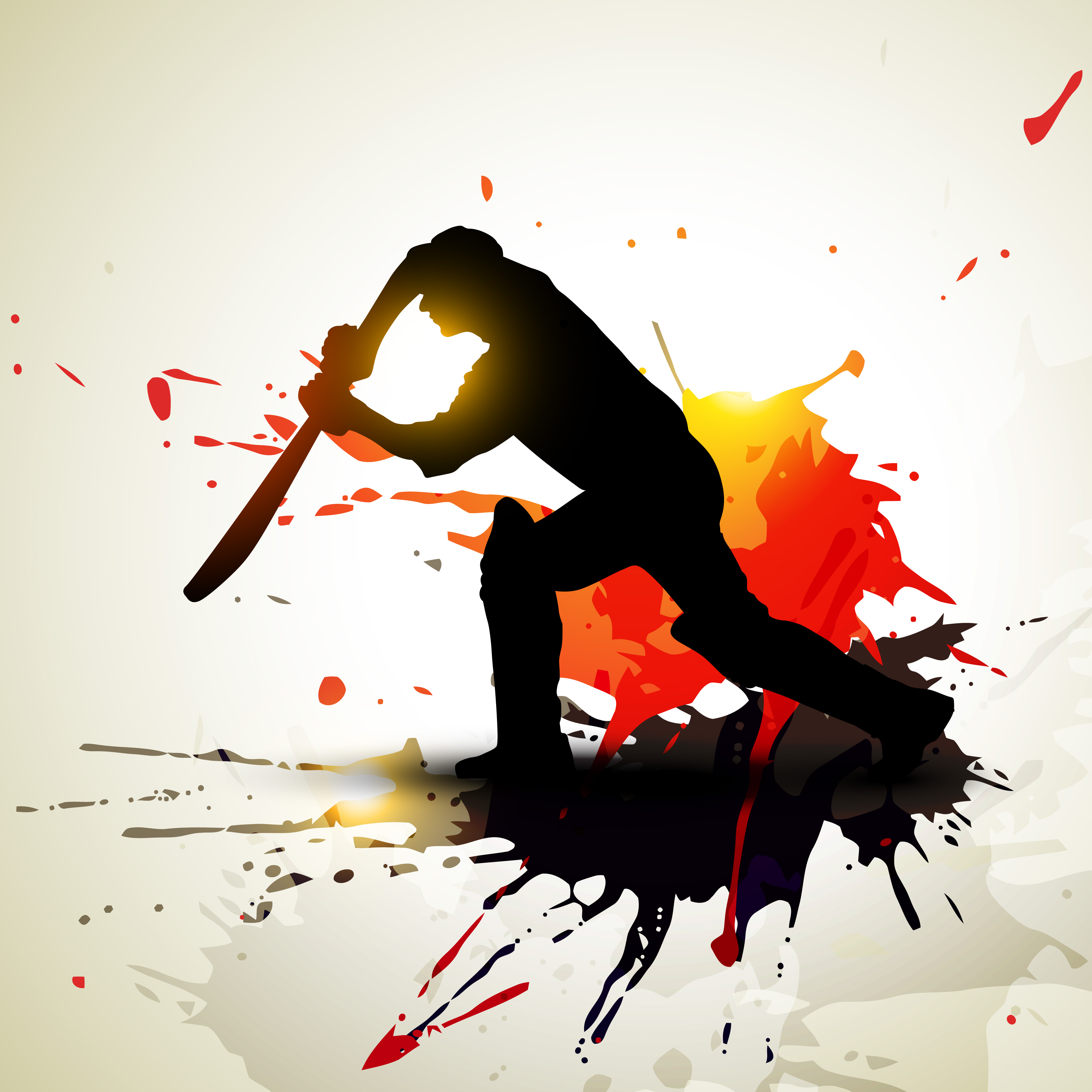The image is a vibrant, modernistic piece of digital art showcasing a deeply shadowed figure in the center. The silhouetted person appears to be captured in a dynamic pose, nearly genuflecting with one leg bent and the other positioned behind them, as if frozen in a moment of intense action. They are grasping a sword or possibly a cricket bat with both hands, extended in front of them, framed by a glowing sun nestled between their arms and casting light between their neck and shoulder.

The artist uses a stark contrast of dark and colorful elements; the figure is rendered in deep blacks and browns, enhancing the sense of shadow and mystery. They wear what might be knee pads or big knee boots, further suggesting a sports player or a warrior-like character. Surrounding this central figure are splashes and splotches of vivid red, yellow, and orange, starkly set against a predominantly white, cream-based background. 

A large, black splotch under the figure's feet and additional speckles and dots around them create a sense of chaos and movement, perhaps symbolizing blood, action, or the remnants of a fierce encounter. The use of colors and abstract shapes throughout creates a dynamic, almost explosive atmosphere, drawing attention to both the silhouetted form in the foreground and the dramatic, colorful landscape behind them.